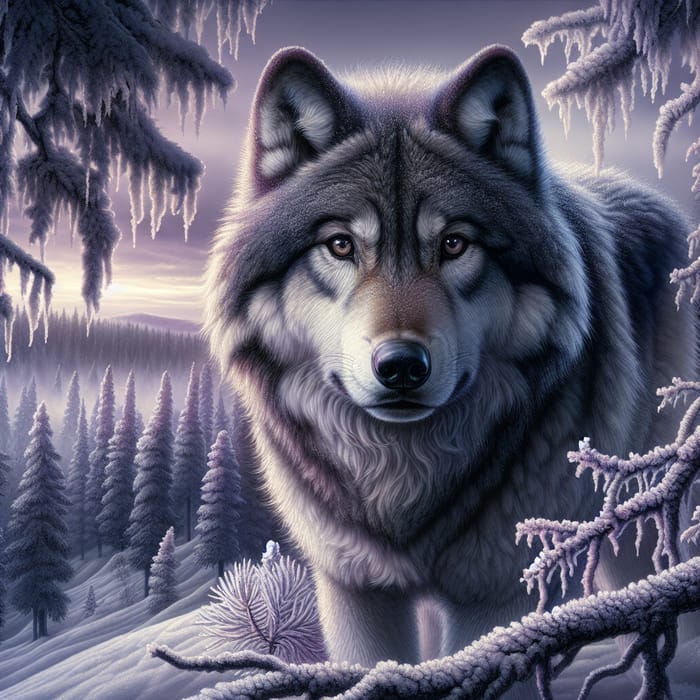This computer-generated pen-and-ink style image depicts a strikingly detailed portrait of a wolf standing in a winter forest. The wolf, with its fuzzy ears and furry coat, is the central focus, captured in a close-up view that makes it seem within arm's reach. Its penetrating gaze is accentuated by deep gray or brown eyes that stare directly at the viewer, above a black nose with subtle brown markings on the snout. The monochromatic scene is enriched with shades of black, white, and gray, punctuated by the wolf's facial details. 

In this snowy landscape, bare branches coated in ice crystals and a sprout of foliage frame the wolf, creating an intimate yet wild setting. Surrounding the wolf are snow-laden evergreen trees and pine needles, from which icicles dangle. The background extends into a distant view of a mountainside, dotted with snow-covered pine trees and silhouetted against a cloudy gray sky. The overall scene exudes a serene, stoic atmosphere, capturing the essence of winter in the wilderness.